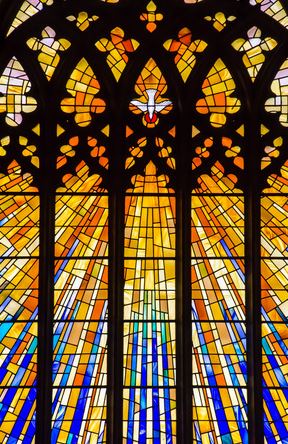This photograph features an elaborate and vibrant stained-glass window, its intricate design housed within a heavy black framework. The window's upper section is dominated by overlapping arches segmented with bisected circles, supporting the intricate glass work beneath it. Four thick vertical black bars run from top to bottom, intersected by thinner horizontal bars forming a sophisticated grid-like pattern.

Central to the top arch is a striking depiction of a white dove, holding a red item in its beak, set against a background of segmented golden glass. This image is surrounded by intricate gothic motifs, including dagger-like elements and club symbols that enhance its ornate appearance.

From the dove, radiant yellow and gold glass segments suggest the rays of a sunrise, fading into vibrant oranges and transitioning downwards into rich blues, symbolizing the sky. This gradient of colors is meticulously pieced together with cut panes of varied yellows, whites, and blues, adding to the window's detailed artistry. The overall effect is a harmonious blend of light and color, suggesting a scene where sunlight emanates from the central dove and cascades downward into a serene blue sky. The image is rectangular and vertically oriented, showcasing the full grandeur of this large and colorful stained-glass masterpiece.